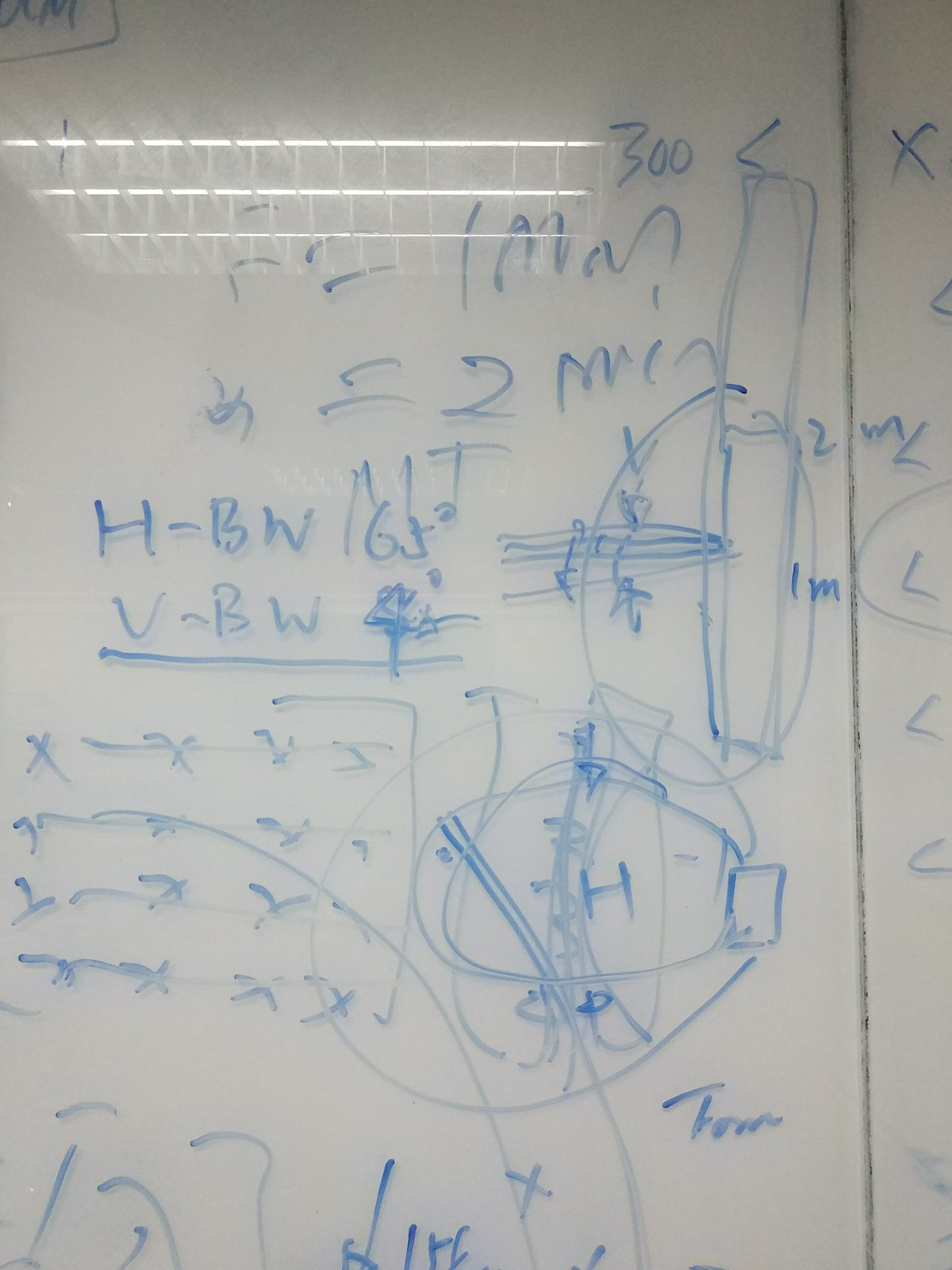This photograph captures a whiteboard that has been extensively written on with a blue marker. The top portion of the board is reflecting a white grid pattern, most likely emanating from an overhead fluorescent light fixture. Covering the whiteboard are various mathematical equations and algebraic scribblings, rendered in very poor handwriting, making much of it difficult to decipher. Among the legible elements, one can identify "300," "X," "F = 1M," "something = 2MIN," "H - BW," "V - BW," "4 degrees," a horizontal line, "X - X," and a partially visible square root symbol. The chaotic scrawl is interrupted by what appears to be random doodles, as if a child had whimsically drawn over the preexisting mathematical notations. The overall scene reflects a cluttered and disorganized attempt at solving math problems, intertwined with playful, distracting sketches.